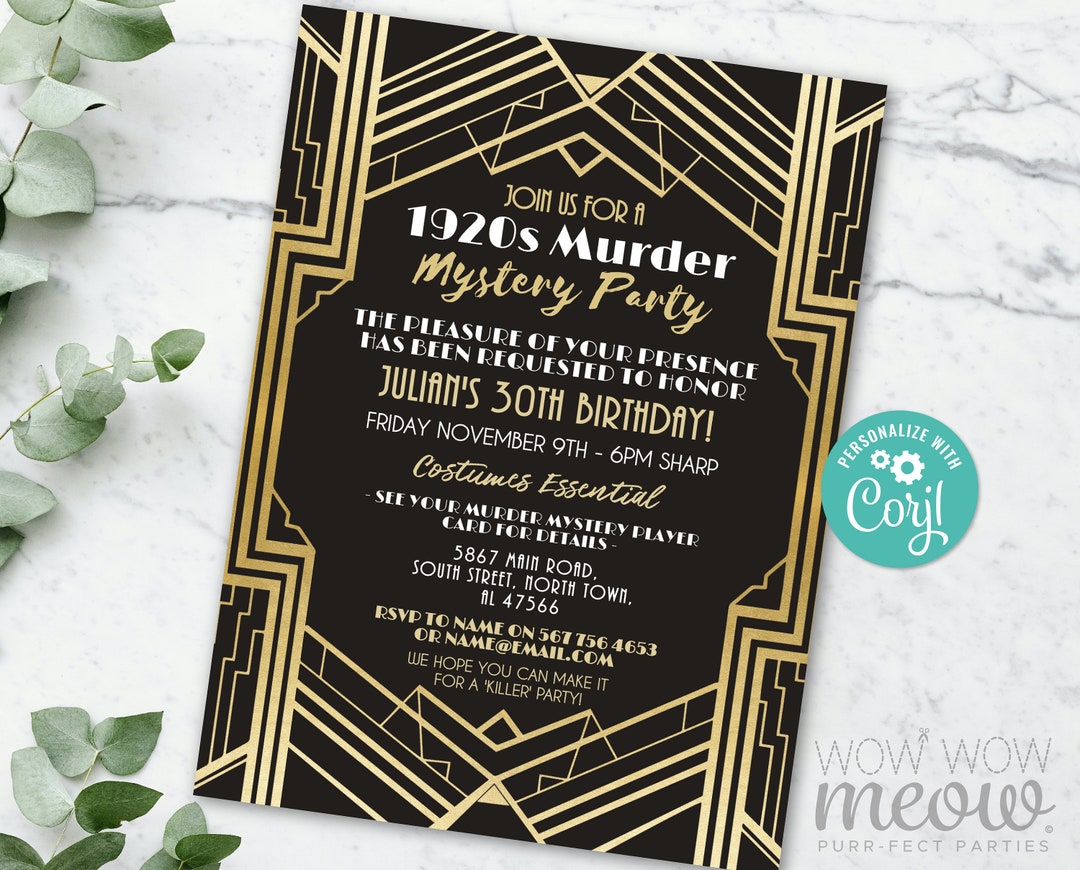The image depicts an invitation to a themed event, set against a marble-like background with green artificial leaves on the left side. A small blue circle on the right boasts the word "personalized" in coral text. In the bottom right corner, the phrase "wow wow meow perfect parties" is elegantly inscribed. 

Centrally featured and slightly tilted to the right, the invitation itself is bordered by gold geometric patterns. Its background is black, providing a striking contrast. The text reads: "Join us for a 1920s Murder Mystery Party. The pleasure of your presence has been requested to honor Julian's 30th birthday, Friday, November 9th, 6 p.m. sharp. Costumes essential. See your Murder Mystery player card for details." It continues, listing the address and RSVP information, inviting guests to confirm their attendance.

The invitation concludes with an enticing promise: "We hope you can make it for a killer party." The gathering promises a thrilling experience, reminiscent of past events where guessing the murderer added to the excitement.